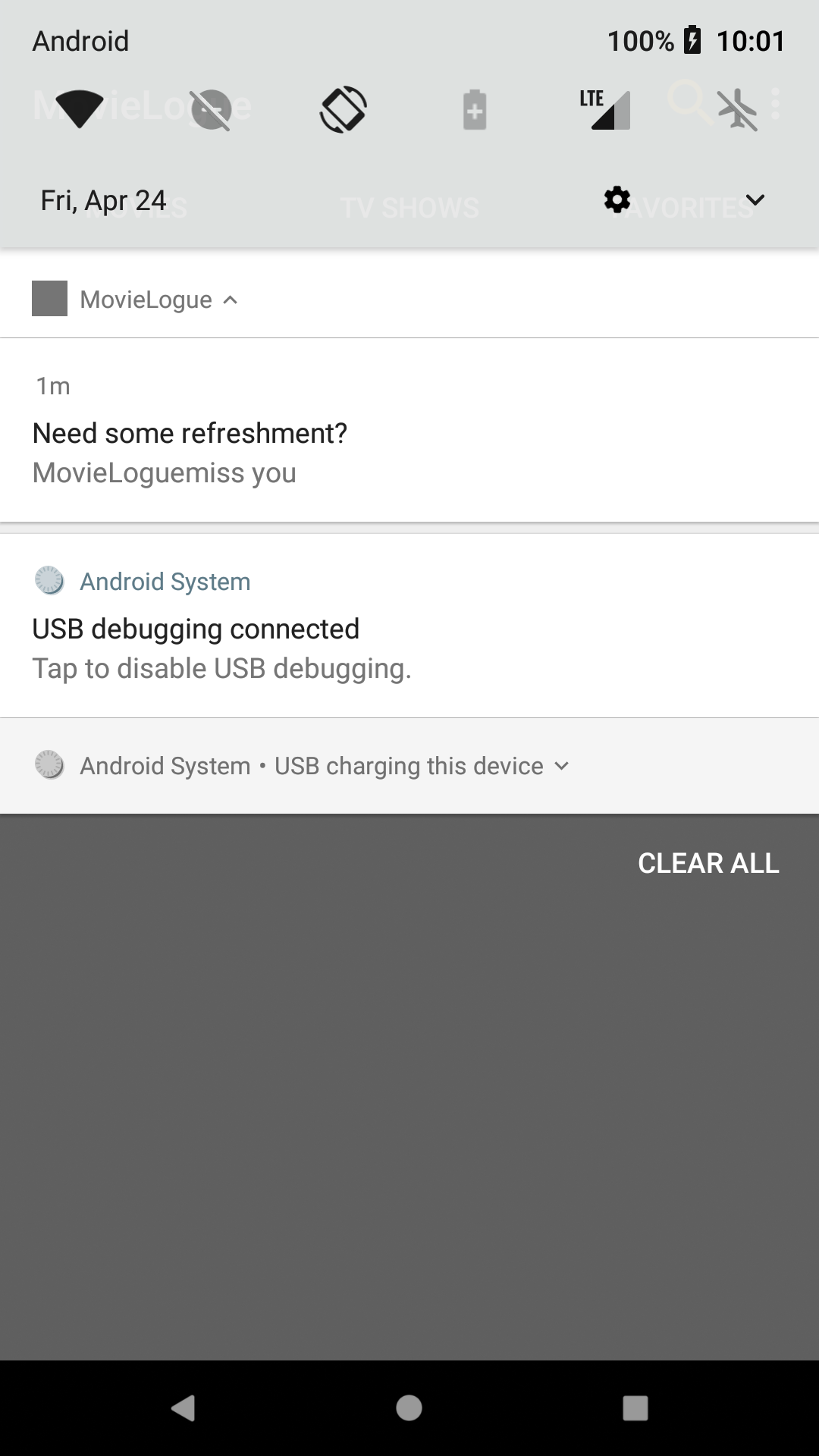A detailed screenshot is shown of an Android smartphone’s notification panel. At the top, the status bar displays various indicators: Wi-Fi is disconnected, Do Not Disturb mode is active, battery level is at 100%, time is 10:01 AM, LTE signal strength, and a search icon resembling a magnifying glass. Directly below the status bar is the current date, Friday, April 24th.

Further down, several icons represent quick settings: Wi-Fi, Do Not Disturb, Screen Rotation, and Battery Saver. A notification titled "LOGUE" from "Movie" appears at the top of the notifications list, timestamped one minute ago, with a message reading, "Need some refreshments, we miss you." Below that, a notification states "USB debugging connected," and offers an option to "tap to disable USB debugging."

Another notification from the Android System indicates "USB charging this device." At the bottom of the panel, the navigation buttons for back, home, and recent apps (represented by a square) are shown, along with an option to clear all notifications. This typical layout provides quick access to essential information and settings, facilitating easy management of notifications.